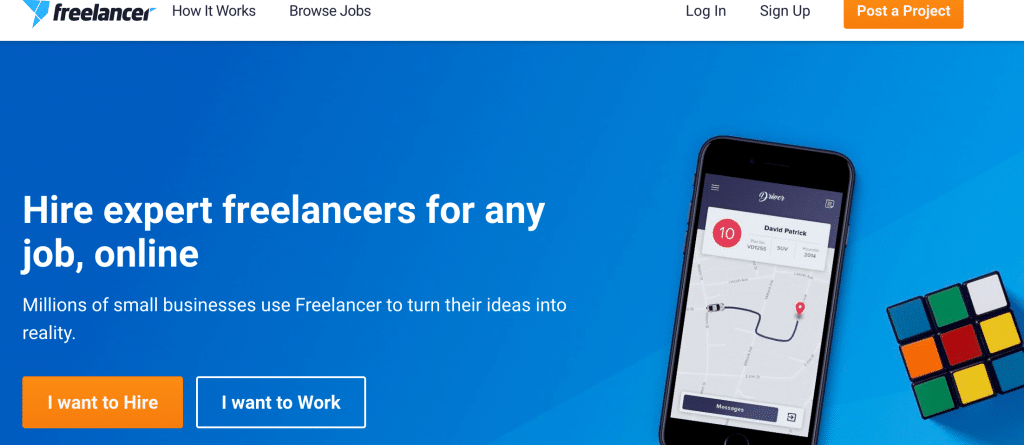The image portrays the top part of a web page with a stark white background that transitions into a blue section toward the bottom. On the top left corner, the word "Freelancer" is displayed in black, accompanied by a blue logo. Moving across the top navigation bar, we see labels such as "How It Works," "Browse Jobs," and other options. On the top right, buttons for "Login" and "Sign Up" are prominently displayed, alongside an orange "Post a Project" button.

The central focus of the page features a blue background with white text on the left-hand side. The text reads: "Hire expert freelancers for any job online. Millions of small businesses use Freelancer to turn their ideas into reality." Below this text, there are two primary action buttons: an orange button labeled "I want to hire" and a standard blue button labeled "I want to work."

On the right side of the image, there's an illustration of a smartphone screen. The screen shows a ride or transport application where a car is traveling to a location marked by the label "David Patrick 10." At the bottom of the app interface, it says "Messages." Additionally, a detailed Rubik's Cube, showcasing its colorful facets of white, green, blue, red, yellow, and orange, is located in the bottom right corner of the page.